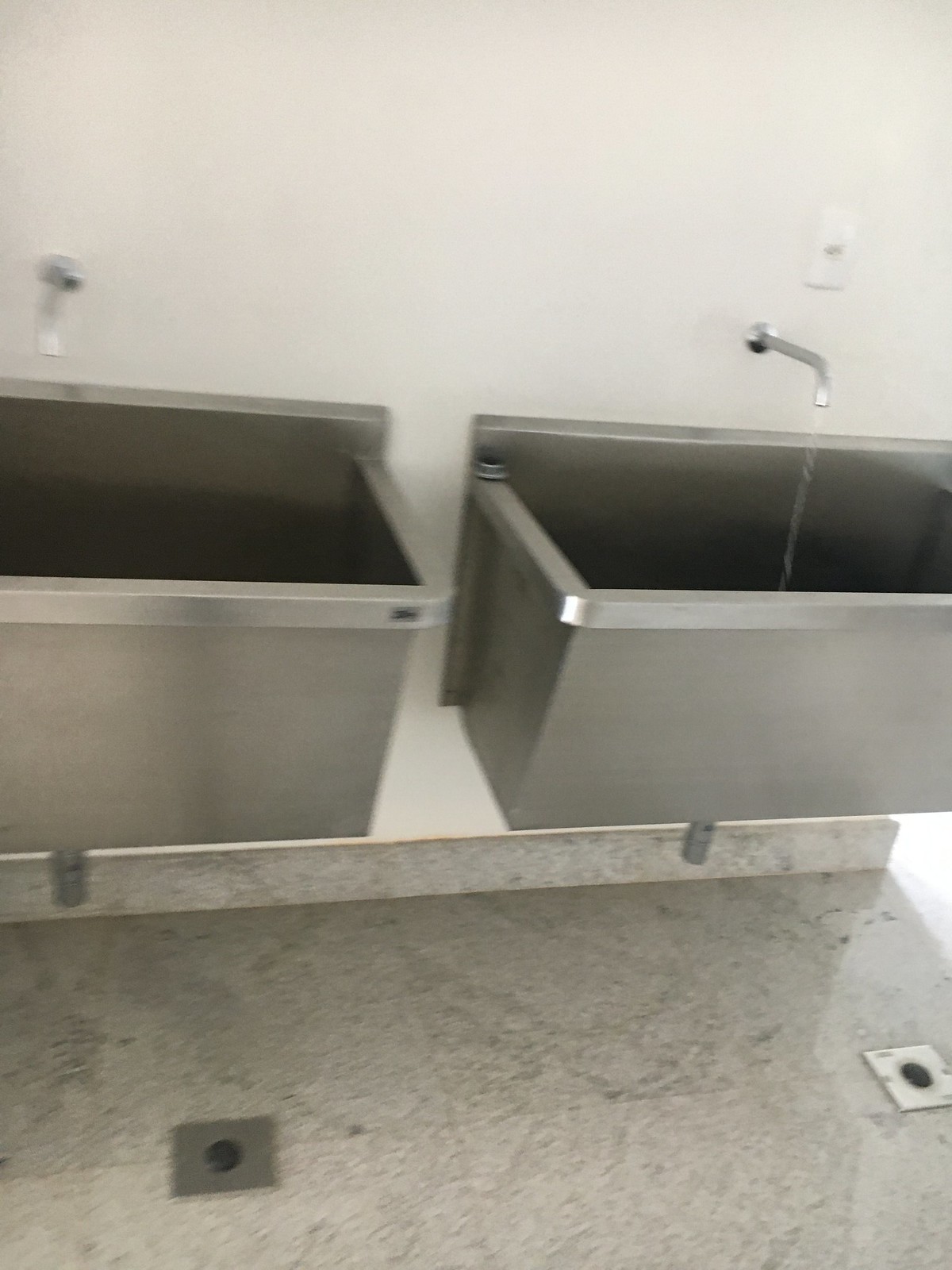The black and white image depicts a stark, utilitarian room with a prominent, clean, white wall. Affixed to the wall are two large, industrial-style sink basins made of silver metal. Each basin is connected to a simple faucet emerging directly from the wall above it, without any handles. Notably, the right faucet is actively dispensing water into the basin below, while the left one remains off. Above the right faucet, a white light fixture and a light switch are visible.

The floor beneath the sinks is covered in white tile, which appears somewhat dirty and marked with black stains, adding to the rugged ambiance of the room. A marble-like baseboard runs along the junction of the floor and the wall. The floor also features two square drain holes, one in front of each sink. The drains are encircled by a silver plate with a black center, providing a functional and straightforward drainage solution in this plainly designed yet practical space.